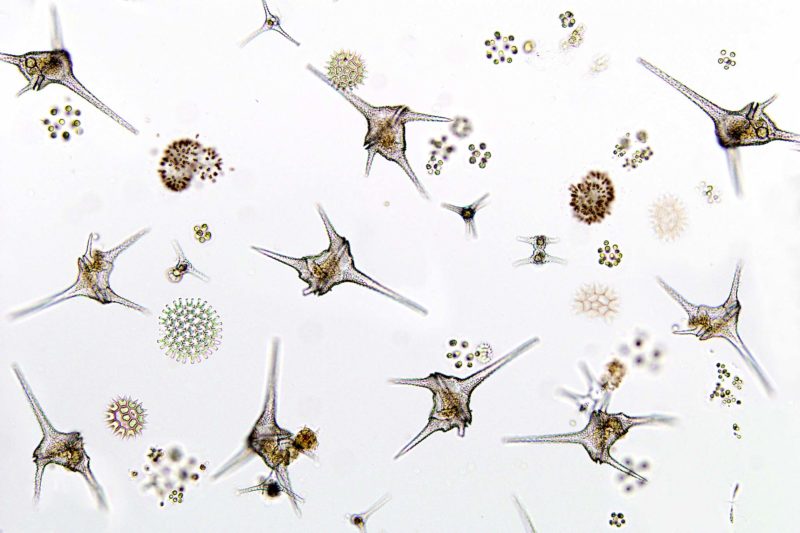The image, in landscape mode, features a cream-colored background filled with intricate digital drawings resembling various forms of microorganisms, possibly bacteria. Dominating the illustration are around eleven white, dandelion-like bursts, accented with green and white details, that appear to represent viral structures or spores. Interspersed among these are clusters of objects in light brown and gray hues, some of which have a distinct, spiky appearance, reminiscent of pointed branches or abstract shapes with sharp edges. Scattered throughout the scene are small dots in shades of brown and green, adding to the sense of diversity and dispersion. The entire composition, though not photorealistic, is meticulously drawn to convey an accurate and detailed representation of microbial life.